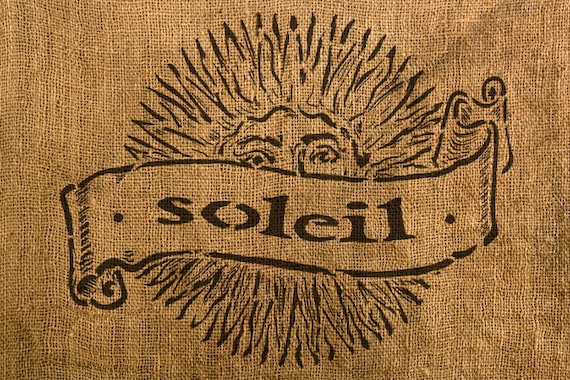This image showcases a detailed, horizontally-aligned stamp on a large beige or brown burlap sack, which is woven with a visible texture. The main focus of the image is a vintage or vintage-style black-ink stamp of a sun with wavy, soft rays forming a perfect circle around it. The sun has a face with detailed eyes and eyebrows visible, but its mouth is obscured by a banner. This banner curls elegantly across the sun's face, revealing shadows that enhance the three-dimensional illusion. In the center of the banner, in lowercase black letters of a serif font that may resemble Times New Roman, is the word "Soleil," flanked by black dots on either side. The word "Soleil," which is French for "sun," stands out prominently against the intricate background of the burlap fabric. The entire composition strikes a balance between a stylized artistic piece and a professional logo, positioned perfectly in the center of the frame.